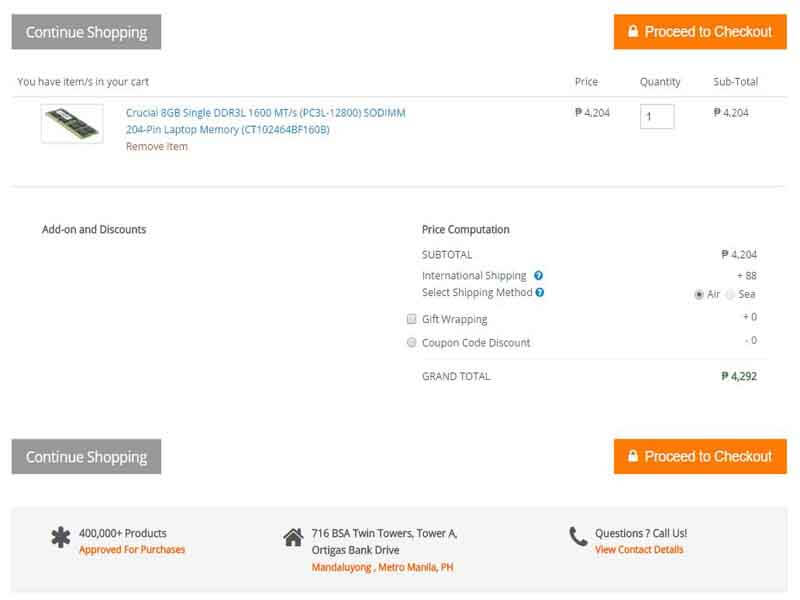This image depicts a checkout page from a shopping website. On the left side of the page, there is a gray button labeled "Continue Shopping." On the right side, an orange box labeled "Proceed to Checkout" is displayed, featuring a lock icon for security. 

Above the cart items section, there is a message stating, "You have items in your cart." The cart includes one item: a laptop memory module, with its quantity mentioned as one. Additionally, there is an accompanying picture of the laptop memory. 

Below the cart, on the right side, a box highlights "Add-on and Discounts." On the left side, the pricing breakdown includes the subtotal, shipping costs, gift-wrap options, coupon code discounts, and the grand total. At the bottom of the page, there is again the orange "Proceed to Checkout" box along with a gray "Continue Shopping" button.